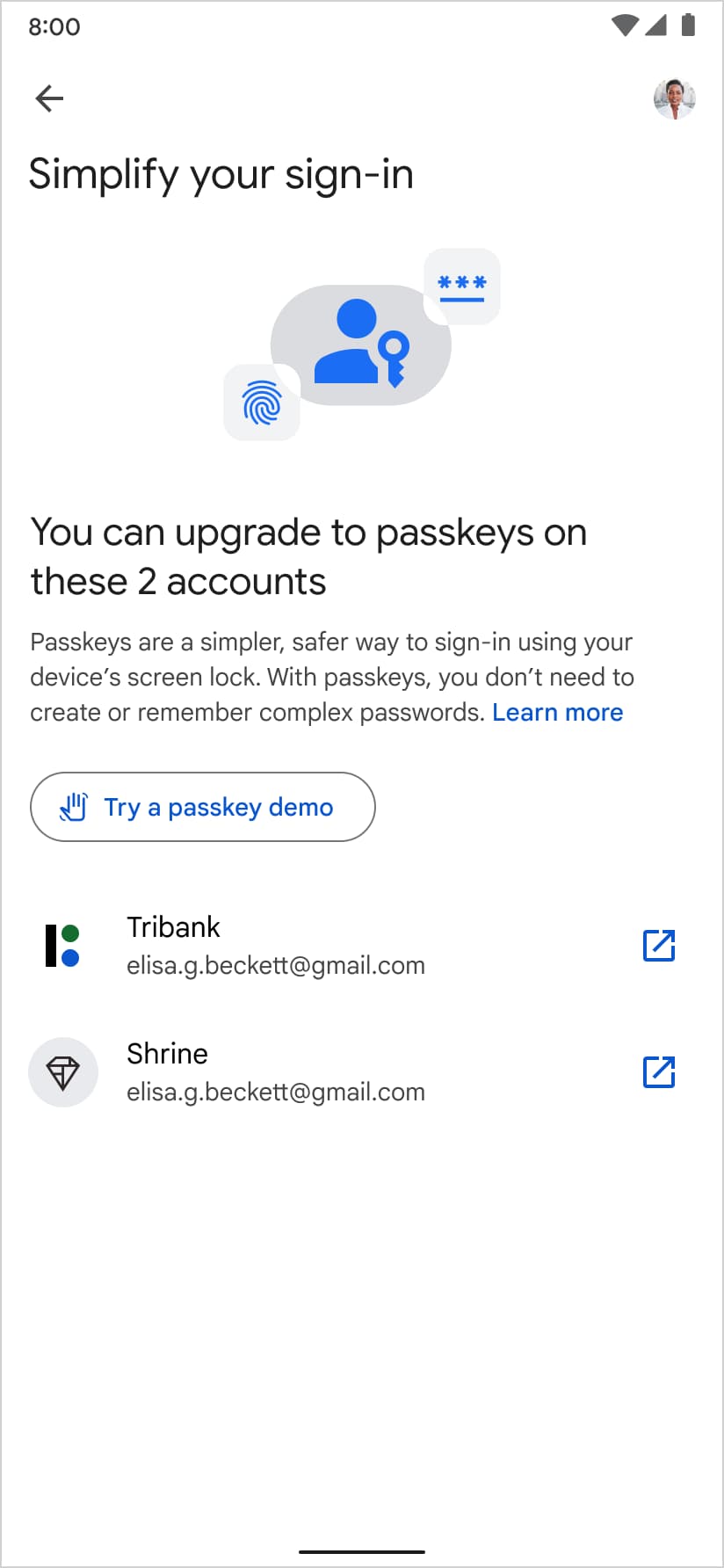The screenshot captures a smartphone's settings interface at 8:00 AM, specifically within a section focused on streamlining the sign-in process. The header reads "Simplify Your Sign-In" and it prominently displays three icons: a fingerprint, a user account with a key, and an emblematic password represented by three asterisks over an underscore. Below this, the text suggests upgrading to passkeys for two accounts, explaining that passkeys offer a simpler and safer alternative for sign-ins by utilizing the device's screen lock, thus eliminating the need to create or remember complex passwords. A "Learn More" link and a "Try a Passkey Demo" button are visible at the bottom, implying an option to explore or simulate passkey usage. The two accounts mentioned are affiliated with TriBank and Shrine, both sharing the same email address.